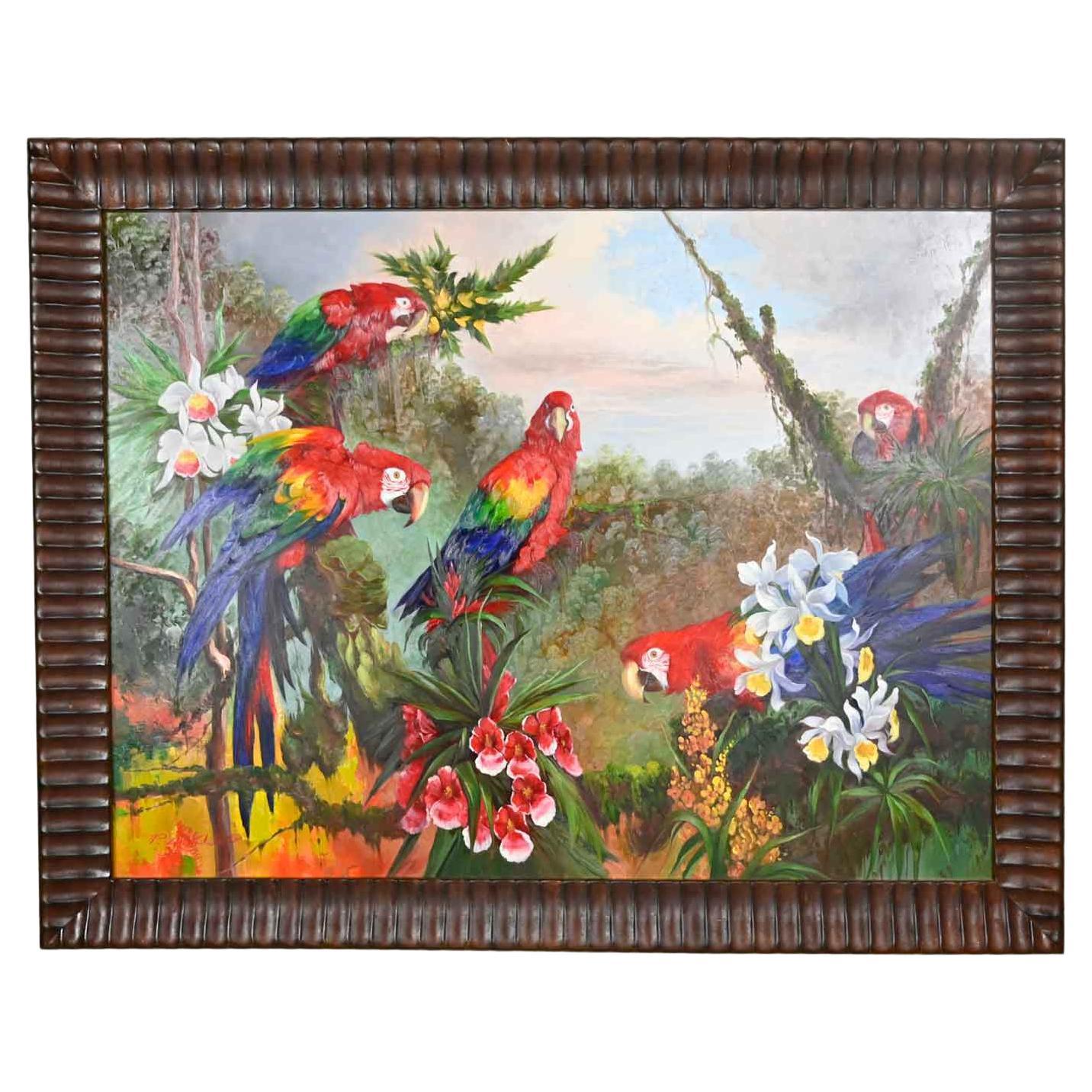This detailed image showcases a framed painting set against a white background, held by a decorative brown frame with textured ridges. The vivid scene within depicts a tropical paradise teeming with five colorful parrots, perched on various trees amidst abundant greenery. These parrots display a striking palette of red, gold, green, and blue feathers, with vibrant orangey beaks and distinctive white rings around their eyes. Central to the composition, one bird gazes directly forward, creating a captivating focal point. The lush environment is further adorned with a rich array of tropical flowers: clusters of white and yellow blooms, pink and red blossoms, and elegant white orchids. The background hints at a misty distance, possibly an ocean or sky, adding depth with its cloudy atmosphere and touches of blue. This intricate painting vividly conveys the beauty of tropical flora and fauna, offering an immersive visual experience.